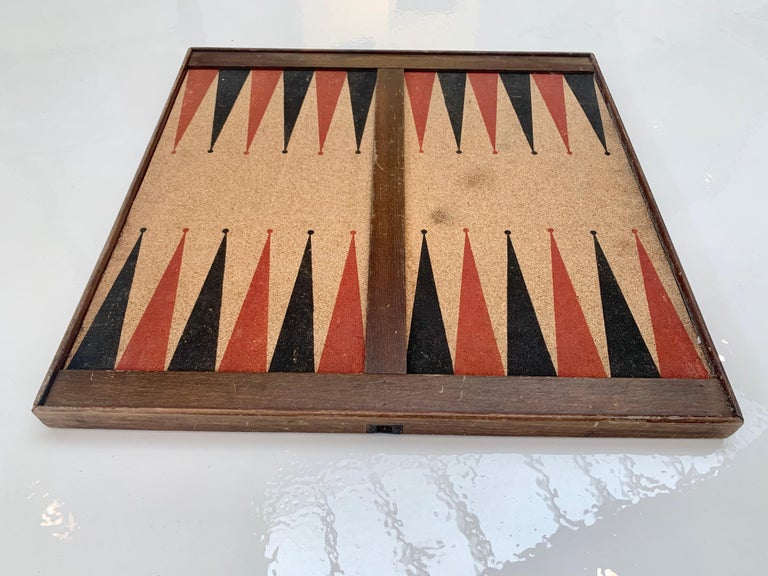The image depicts a detailed wooden backgammon board resting on a shiny, white table. The board is square in shape with dark wooden framing and a prominent wooden divider running vertically down the center. The playing surface has a light brown or cork-like texture, and both the top and bottom sections feature a series of alternating red and black triangles, known as arrows or darts. Each triangle is tipped with a small ball. The board is displayed in a landscape orientation, giving it an old-fashioned appearance. The table beneath the backgammon board is starkly white, creating a striking contrast with the game's vibrant design.